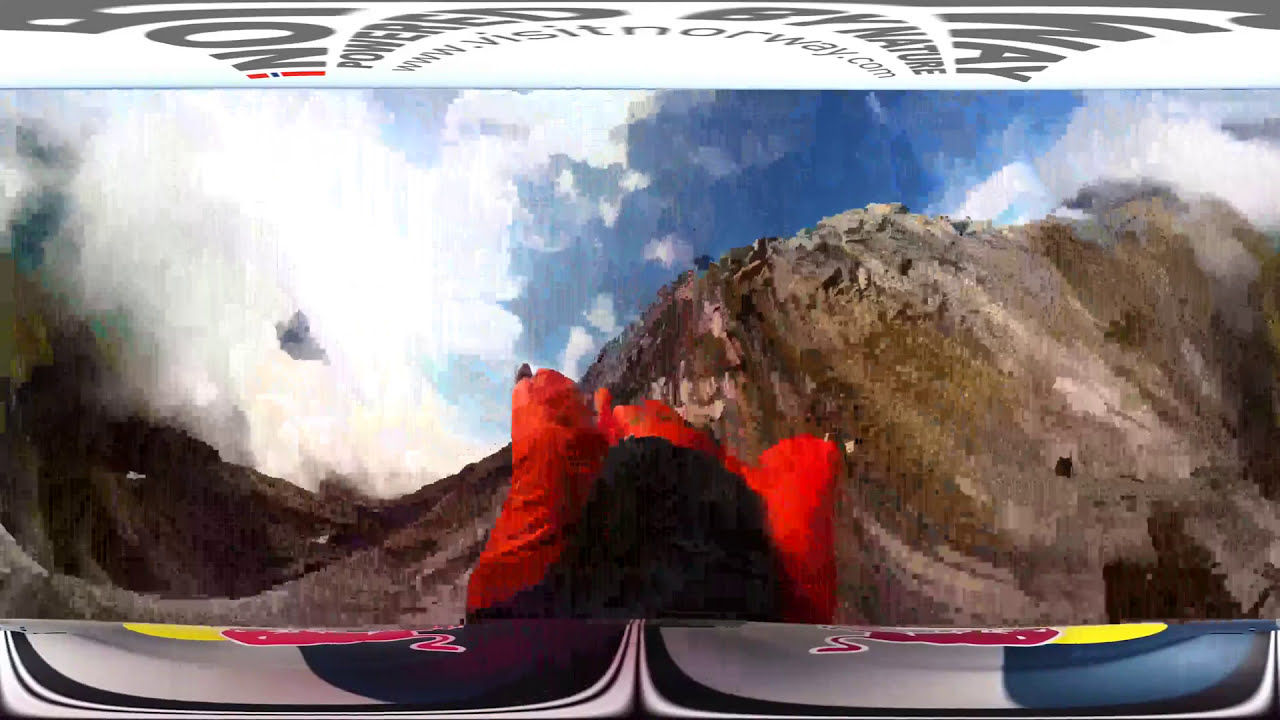The image is a very low-resolution photograph, likely around 240p, depicting a person in a red and black suit seemingly engaged in hang gliding or skydiving above a mountainous region. The suit appears designed for wind resistance. The backdrop showcases a brown, possibly gray-tinted mountain, with a vibrant blue sky and white clouds, which are described as slightly dusty on the left. Central to the image is the person wearing the suit, surrounded by the expansive sky and mountainous terrain. At the top of the photo, there is stretched-out text reading "visit Norway dot com," though it's slightly obscured and stretched. Some viewers also noted additional elements like potentially photoshopped sections and a possible reference to Red Bull with its iconic red and yellow colors. The overall impression is of an adventurous scene captured in a scenic, albeit blurry, outdoor setting.